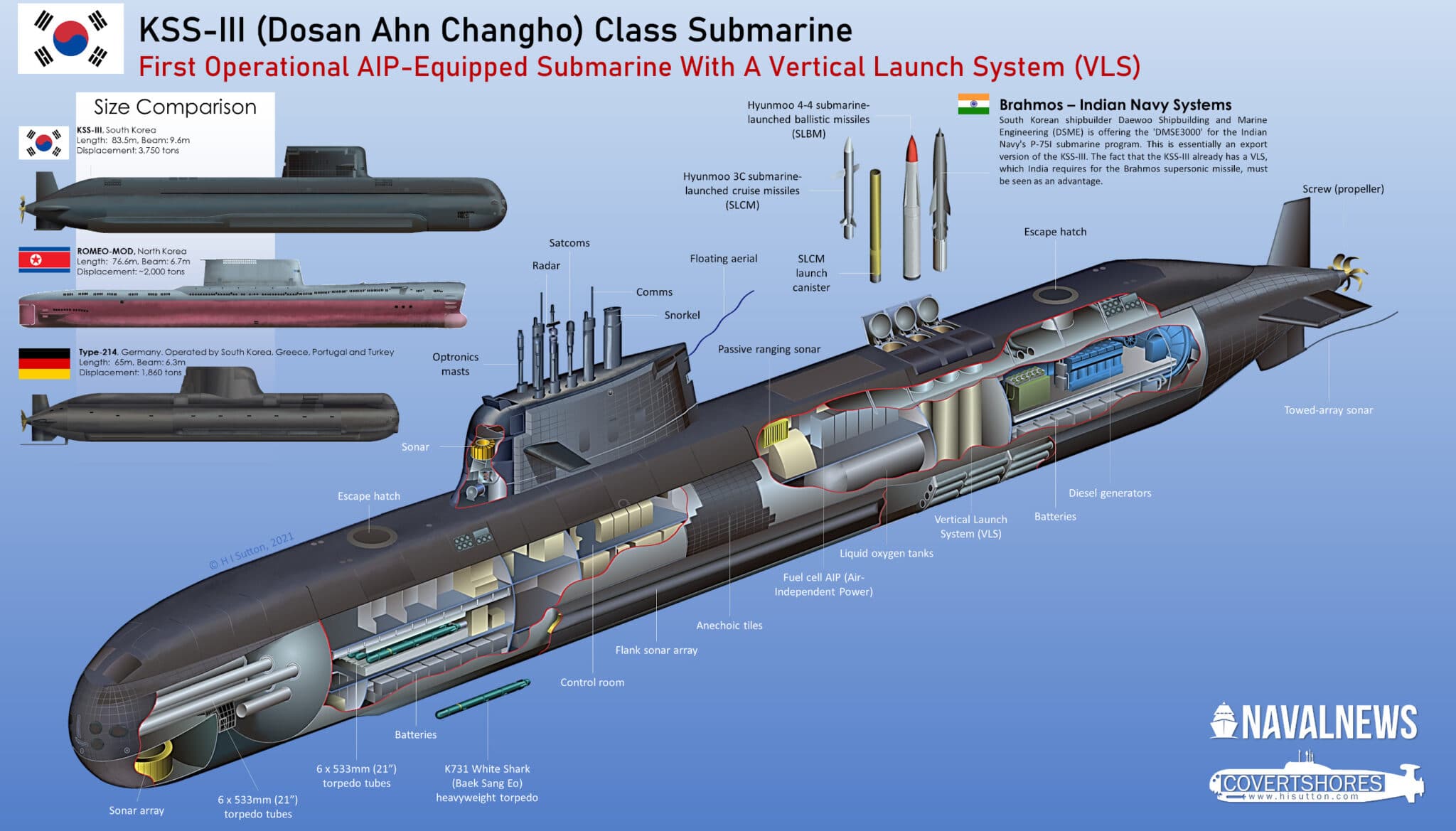The image is a detailed technical illustration of the KSS-III (Dosan Ahn Changho class) submarine, prominently featuring the first operational Air-Independent Propulsion (AIP) equipped submarine with a Vertical Launch System (VLS). The centerpiece is a cutaway view showing the internal compartments, each labeled in black and white text. A South Korean flag is positioned in the upper left corner. Naval News branding appears in the bottom right corner, accompanied by a submarine icon with blue and white lettering. The upper right side identifies the submarine in red text and highlights it as the "First Operational AIP-Equipped Submarine with a Vertical Launch System." Below that, there is information about various missiles that the submarine can launch vertically. A size comparison chart on the left features three submarines from South Korea, Germany, and one unidentified country, alongside their respective flags. Additionally, the Bahamas flag and BrahMos Indian Navy systems are noted in the upper right section. The illustration emphasizes the submarine's advanced technology and superior size compared to others.